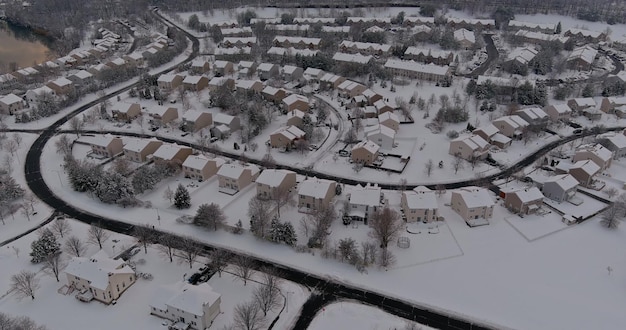The aerial photograph captures a suburban neighborhood enveloped in a blanket of snow, highlighting the quiet uniformity of the landscape. You see a road slicing through the scene from top to bottom and another curving from left to right, intersecting on the left side. To the left of the image, distinct older farmhouses with driveways break the uniformity of the otherwise identical double-decker houses. Trees are scattered throughout, mostly bare and dormant, though a few dark green pine trees stand out. A small lake is visible in the top left corner, surrounded by leafless trees. The overwhelming sense is one of winter stillness, with snow-covered buildings and land, creating a serene yet desolate winter scene seen from a high vantage point.